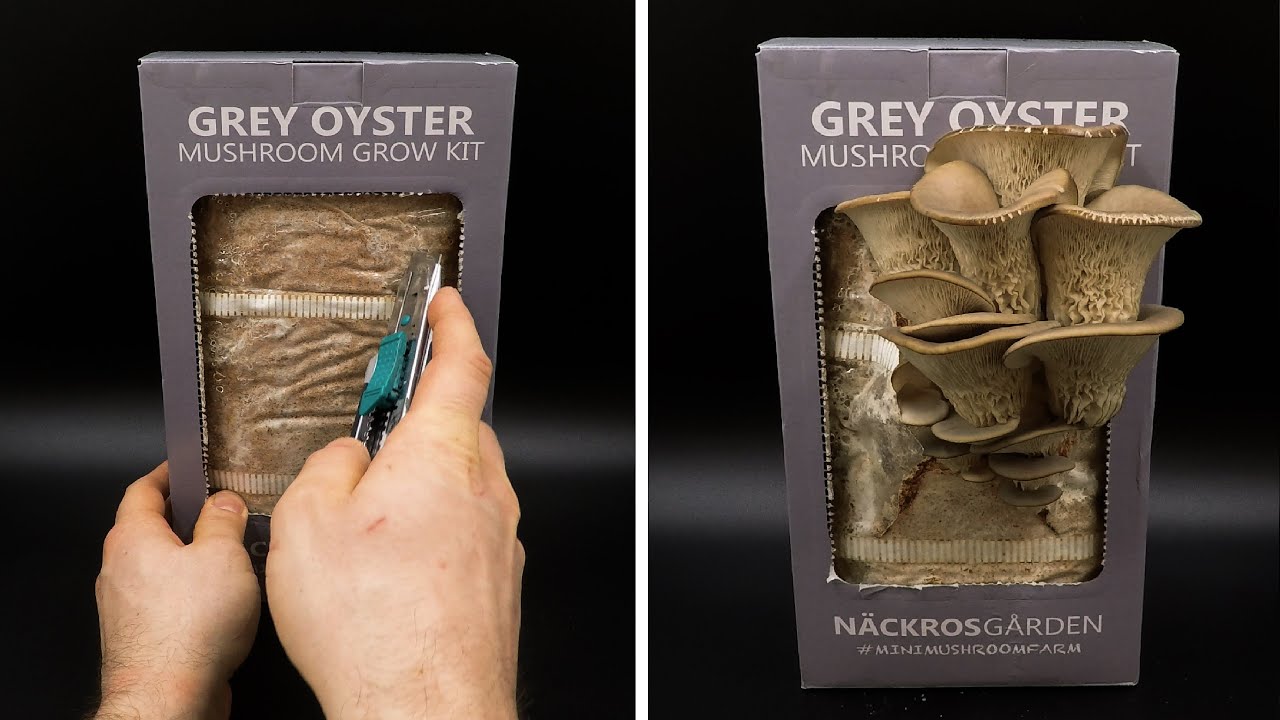The image depicts an advertisement for the Nacrose Garden Great Oyster Mushroom Grow Kit, presented in two photographs against a black background. In the first picture, a person with light skin is shown using a razor blade to carefully cut open the front of a gray box labeled "Gray Oyster Mushroom Grow Kit," and to remove the plastic wrap. The second picture reveals the same box after it has been opened; the plastic has been removed and mushrooms are beginning to sprout from the box. The bottom of the box features the brand name "Nacrose Garden" alongside the hashtag "Mini Mushroom Farm," illustrating the initial and growing stages of the mushroom kit.